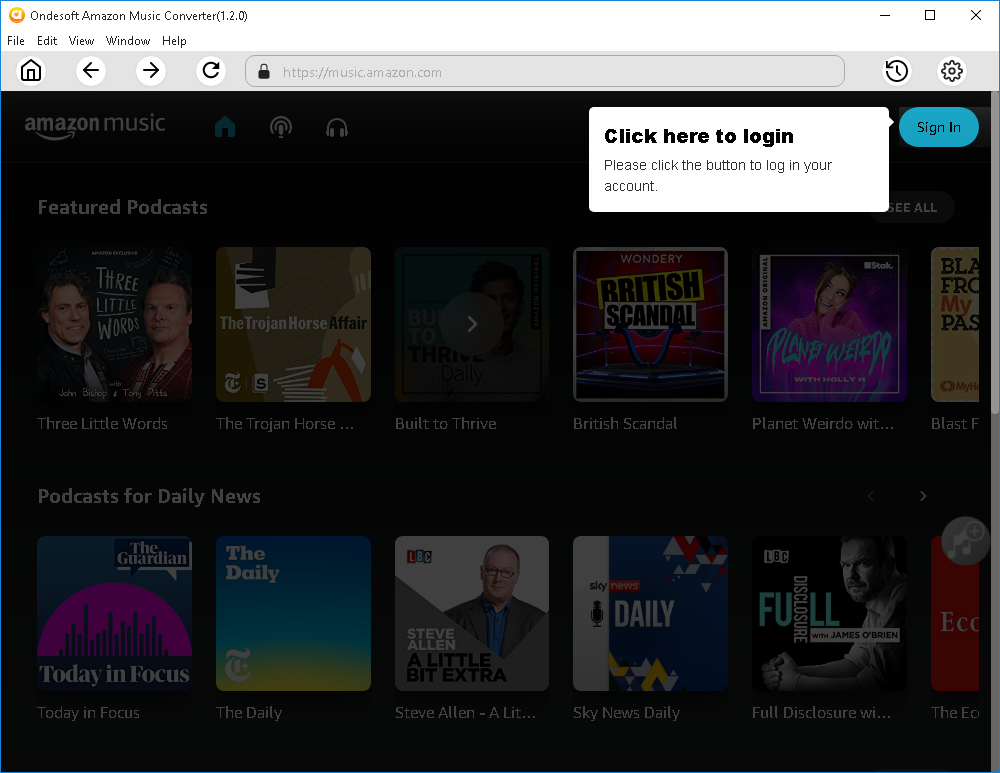Screenshot of the Amazon Music login page with greyed-out sections displaying small thumbnails for various podcasts and news programs. In the top right corner, there is a blue 'Sign In' button with black text. Accompanying the button is a white speech bubble with black text instructing users to "Click here to log in. Please click the button to log in to your account." This appears to be part of a diagram or illustration guiding users on how to log in to Amazon Music.

In the background, the main screen features a blacked-out area with rows of highlighted podcasts. The featured podcasts section includes titles such as "Three Little Words," "The Trojan Horse," "Built to Thrive," "British Scandal," and "Planet Weedo." Additionally, the Daily News podcasts section lists titles including "Today in Focus," "The Daily," "Steve Allen," "A Little Bit Extra," and "Sky News Daily."